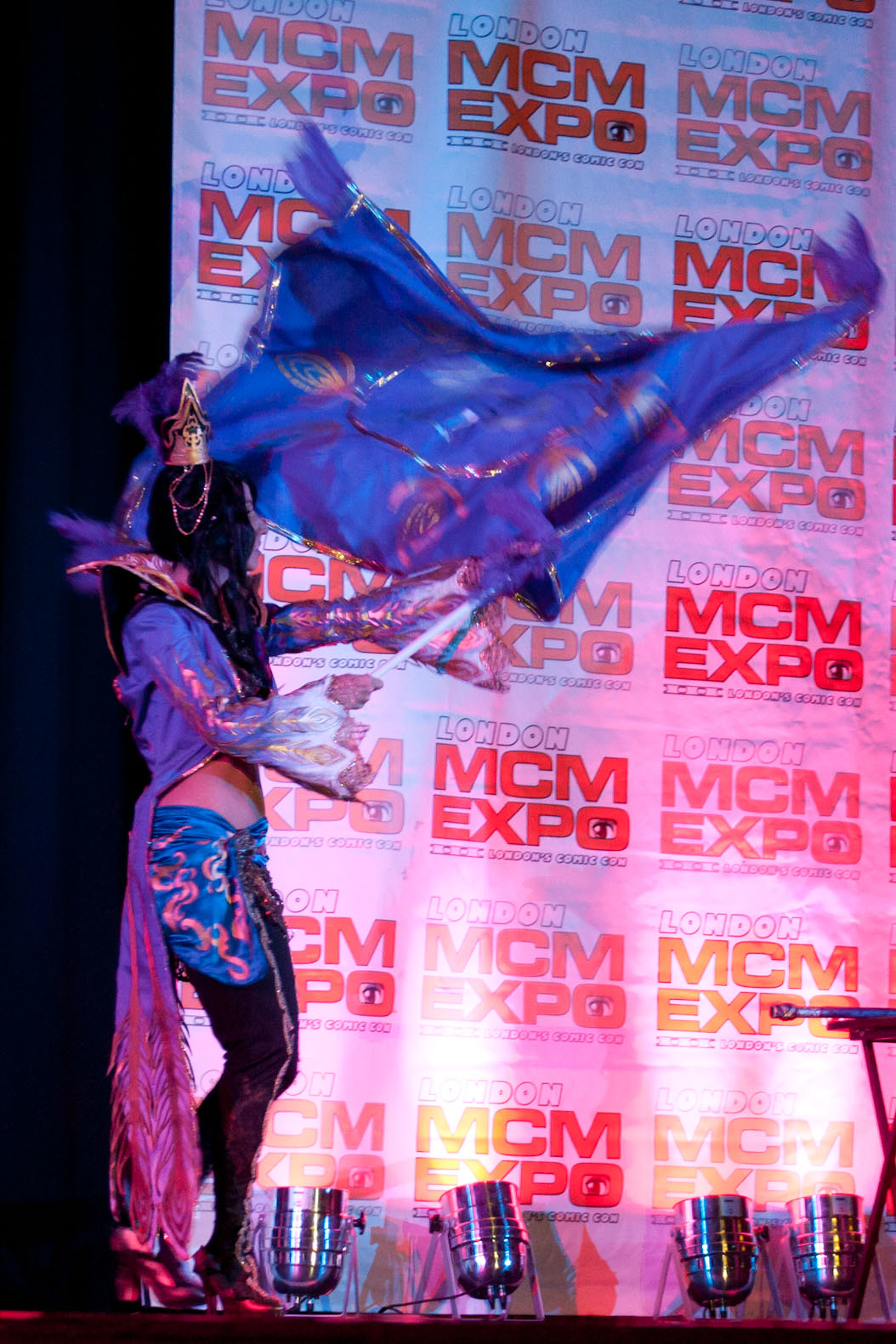This is a detailed photograph capturing a performer on stage at the London MCM Expo. The woman, who appears to be around 30 years old, stands on the left side of a dark indoor stage. She is energetically waving a large blue flag adorned with golden designs. Her elaborate costume includes a long-sleeved blue jacket that transitions into purplish-pink, feather-like tails, paired with a blue and gold skirt, black tights or leggings, and striking red shoes. Atop her head, she wears a golden conical cap which complements her vibrant attire. Behind her, a prominent poster dominates the black background, repeatedly displaying the event's "London MCM Expo" logo. The words "MCM Expo" are boldly written in red letters, with "London" in white above them. The poster features multiple repetitions of the logo in rectangular frames. At the bottom of the stage, silver lights aimed upward illuminate both the performer and the poster, adding a dramatic effect to the scene.